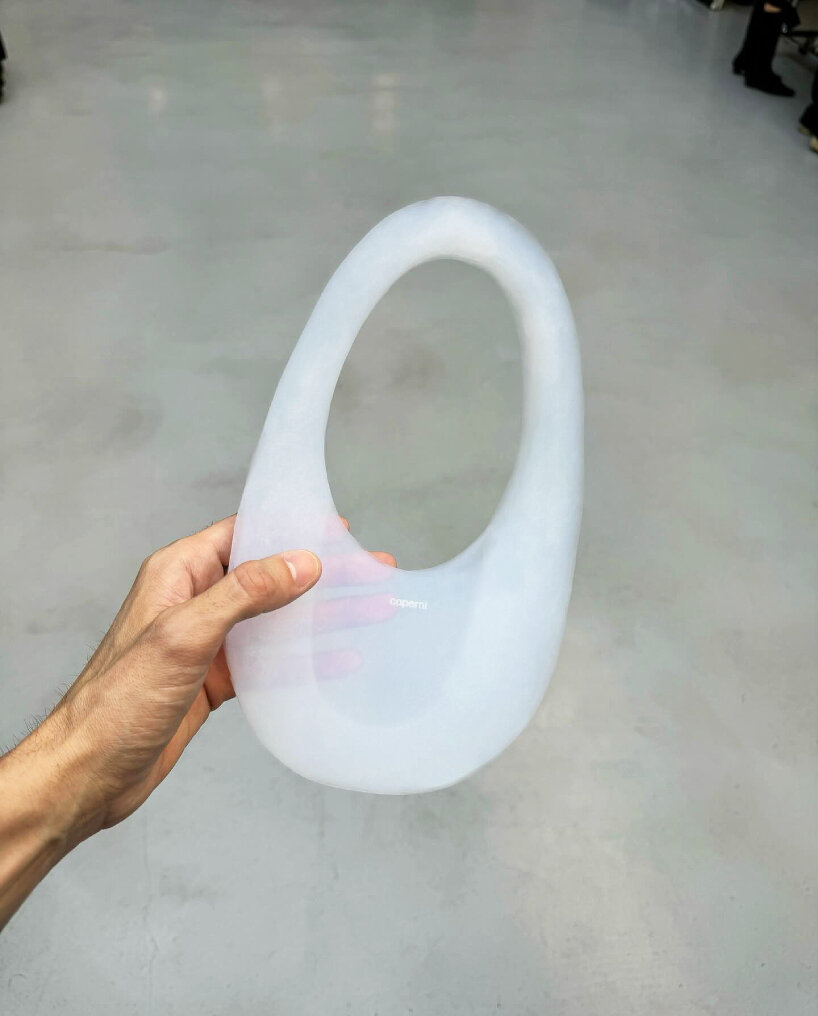In this photograph, a human hand prominently holds a translucent, cylindrical plastic object centrally in the frame, drawing immediate attention. The object has an elongated, egg-like shape and features an oval opening at its top, suggesting it might be a cover or holder of some kind. The material of the object appears cloudy or silverish, contributing to its unique and somewhat mysterious form. The backdrop includes a marbleized floor with light reflections, and in the top right corner, there are feet wearing boots, hinting at a larger, potentially public indoor setting like a store. The overall composition centers around the unusual, semi-transparent plastic item, framed by the subtly reflective and busy background.